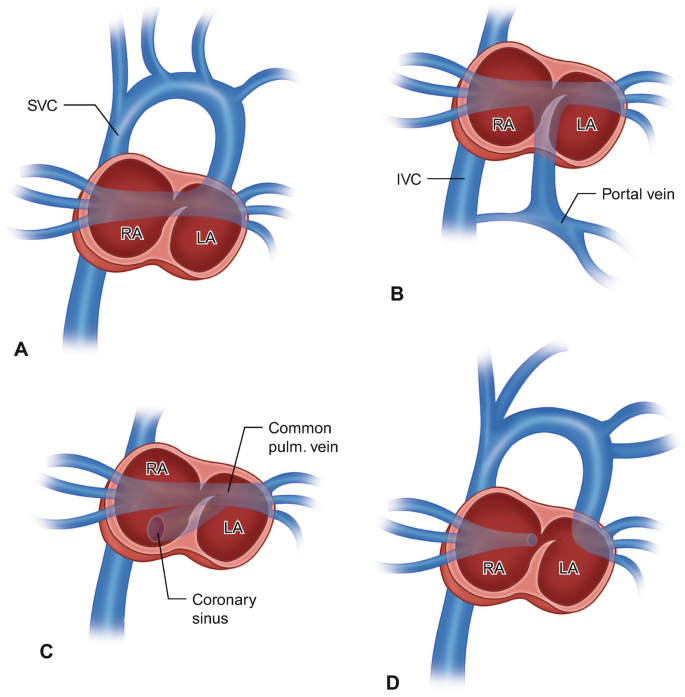This medical diagram consists of four stylized images labeled A, B, C, and D, illustrating various views of veins intersecting with cardiac elements. Each image occupies one quadrant of the overall diagram. The veins are uniformly depicted in blue against a white background, while the red internal structures, containing chambers labeled R, A (right atrium), and L, A (left atrium), form the central focus of each quadrant. In Image A (top left), a single blue vein labeled SVC curves downward into two red chambers. Image B (top right) features the blue vein labeled IVC splitting at the bottom, with an adjoining branch labeled the portal vein, and curving upwards into the red chambers. Image C (bottom left) shows a straight blue vein running through the two red chambers, flanked by another two veins labeled coronary sinus on the left and common pulmonary vein on the right. Image D (bottom right) similarly depicts a curved blue vein flowing into the two red chambers, with labels consistent with those in the other images. This diagram is designed for medical professionals to illustrate the anatomical relationships between these specific veins and the heart chambers.